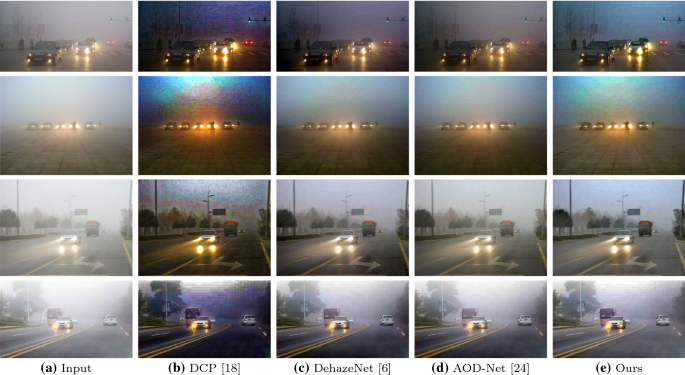This image collage consists of a series of 20 square images, arranged into a larger grid, depicting various scenes of traffic under different conditions. In the first series of images (labeled 'Input' at the bottom), a car is advancing towards the viewer on a very hazy street, creating a foggy atmosphere. In subsequent images within this row, varying lighting conditions and times of day are illustrated, showing how the scene looks in different light scenarios.

The second series of images (labeled 'B, DCI, P, 18') show a similar sequence but with a bluer and more blurred background. As you move to the next row (labeled 'C, D, Haze, Net, 6'), the images become clearer with reduced haze, especially noticeable in the bottom two images of this row. 

In the fourth row (labeled 'D, AOD, Net, 24'), the clarity increases further, akin to the images in row ‘C', but slightly more refined. Finally, in the last series (labeled 'E, Ours'), the images are the clearest, with minimal fog or blurring, showcasing the same traffic scenarios.

Throughout the grid, each traffic situation varies: some images feature multiple parked cars with their headlights directed towards the viewer, while others show moving vehicles and even a bus, all depicted in various degrees of haze to trial different image processing techniques. The detailed annotations at the bottom reference the specific methods applied to each column of images.